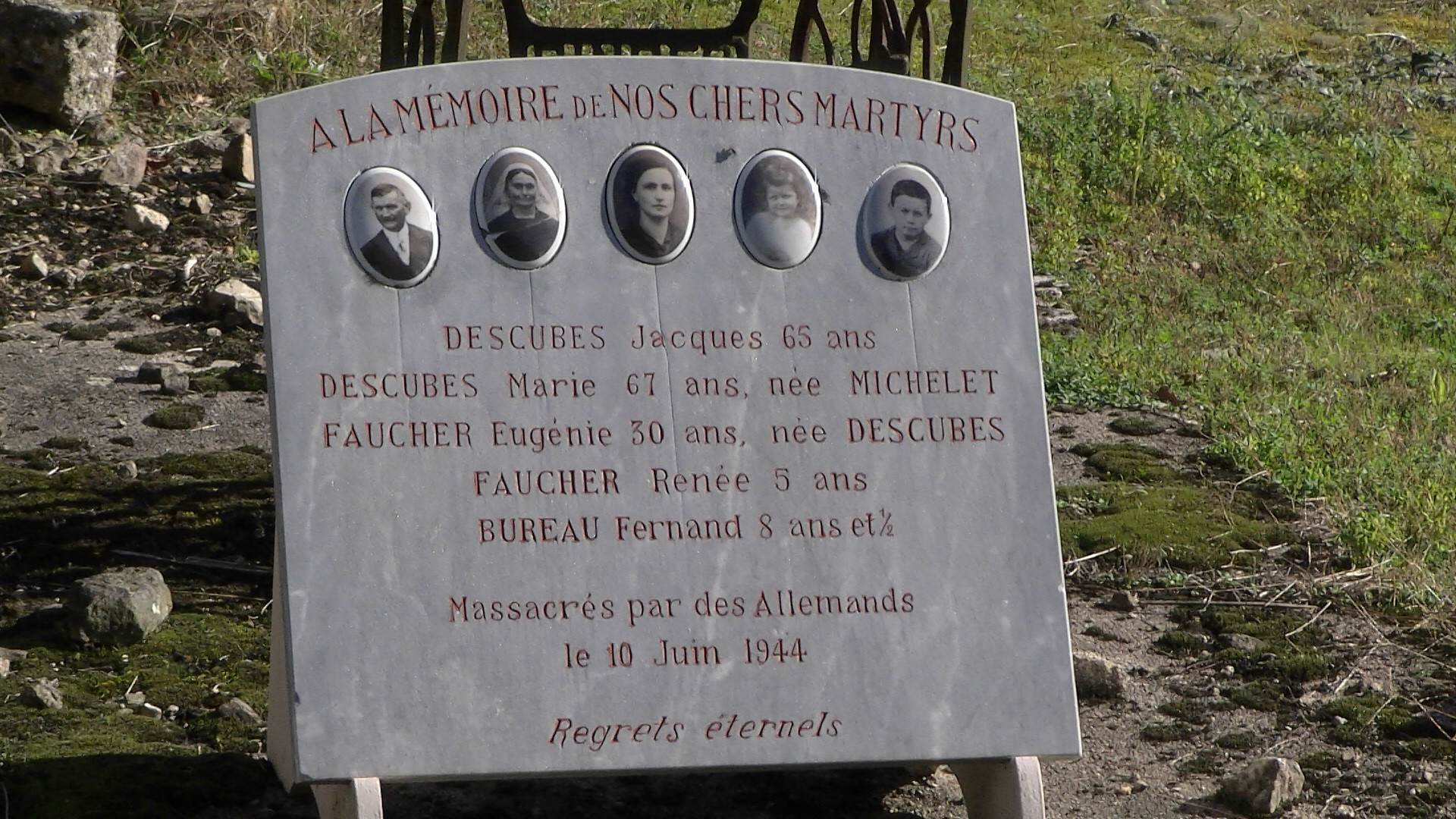This photograph, taken outdoors during the daytime in landscape mode, depicts a gravestone-like stone plaque placed on the ground against a black metal holder. The scene is surrounded by green grass and a rocky pathway. The gray stone plaque bears five oval photographs of individuals. At the top, carved into the stone in red, it reads "A la mémoire de nos chers martyrs," which translates to "In memory of our dear martyrs." Beneath the photos are the details of each person: Jacques Descubes, 65 years old; Marie Descubes (née Michelet), 67 years old; Eugenie Foucher (née Descubes), 30 years old; Renée Foucher, 5 years old; and Ferdinand Bureau, 8 and a half years old. Below this, in French, it states that they were massacred by the Germans ("massacre par les Allemands") on June 10, 1944. This memorial plaque commemorates these individuals, who were among the victims of an atrocity that occurred in France during World War II.